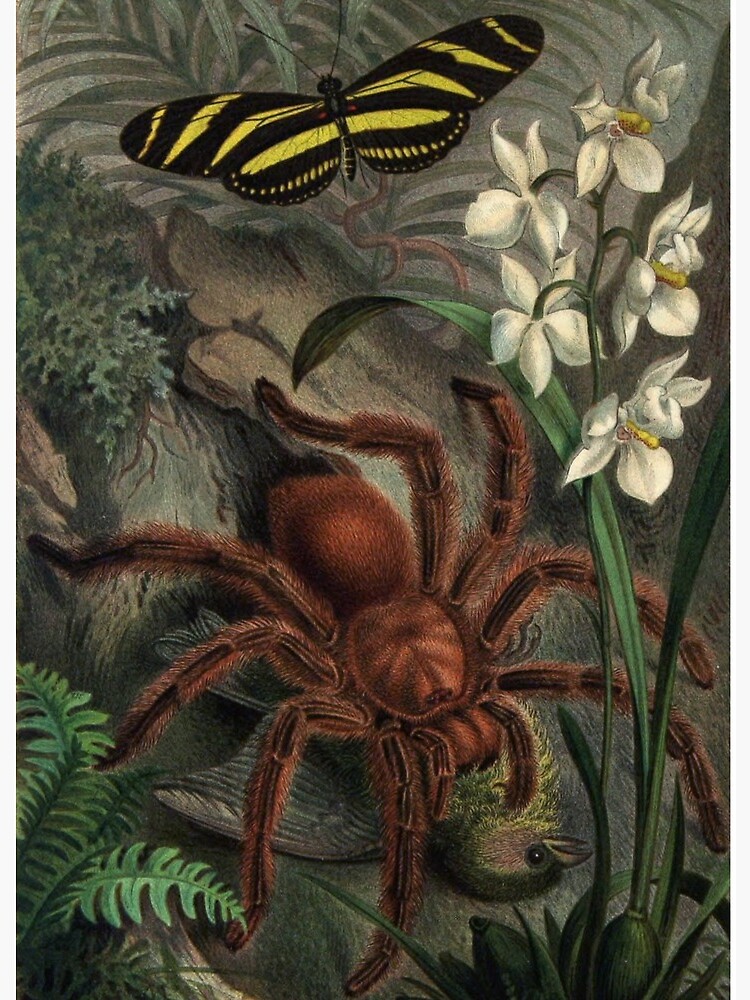The digital illustration presents a detailed outdoor scene featuring a South American goliath tarantula with its brown, hairy body prominently positioned at the center as it devours a vividly colored bird, which mixes greens, yellows, and grays. The scene is surrounded by natural elements, including grass, shrubs, and fern leaves. To the side, a plant with elegant white orchids adds a touch of delicate beauty. Above the tarantula, a striking black and yellow butterfly with tiger-striped wings hovers, observing the tableau from above. The illustration portrays a soft, naturalistic ambiance, rich in both botanical and zoological details.